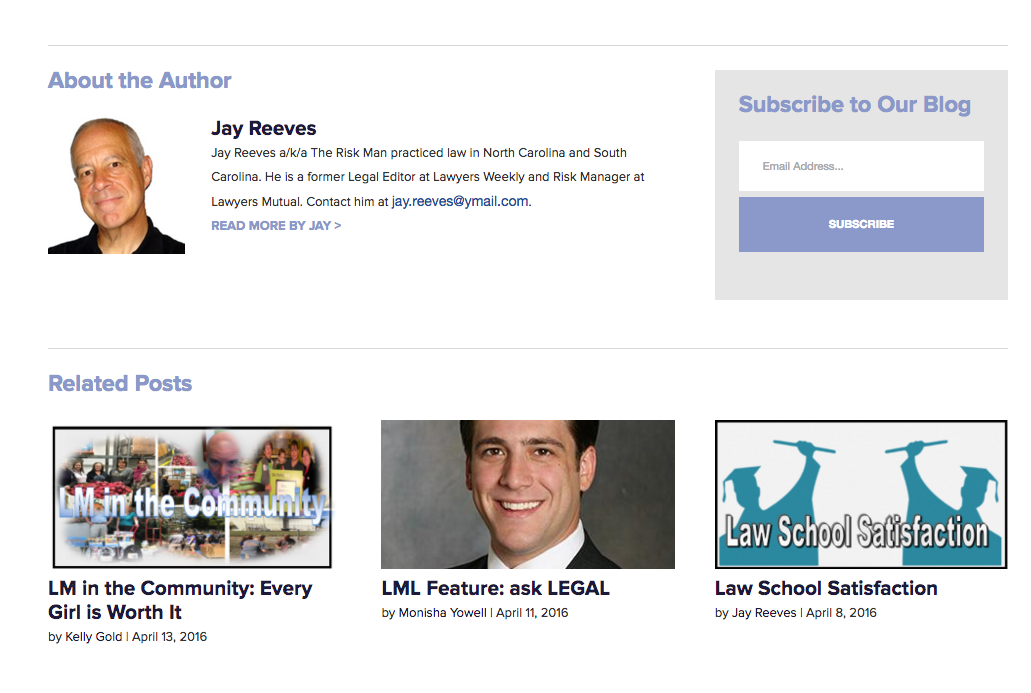**Detailed Caption:**

The image displays a detailed web page about the author Jay Reeves, known as "The Risk Man." Jay Reeves has a background in practicing law in both North Carolina and South Carolina. He is also a former legal editor at Lawyers Weekly and is associated with risk management at Lawyers Mutual. The page provides his contact email as JayReeves@ymail.com. There’s a “Read more by Jay” hyperlink that redirects to a collection of his other writings. Below this, there's an invitation to subscribe to the blog by entering your email address, with a light blue "subscribe" button. Further down, the page lists related posts under titles such as "Law School Satisfaction," "LML Feature Ask Legal," "LML in the Community," and "Every Girl is Worth It," which appear to be advertisements. The highlight of the page is Jay Reeves's author profile, emphasizing his skills as a editor and legal professional, attracting visitors to learn more about his work and contributions to the field.